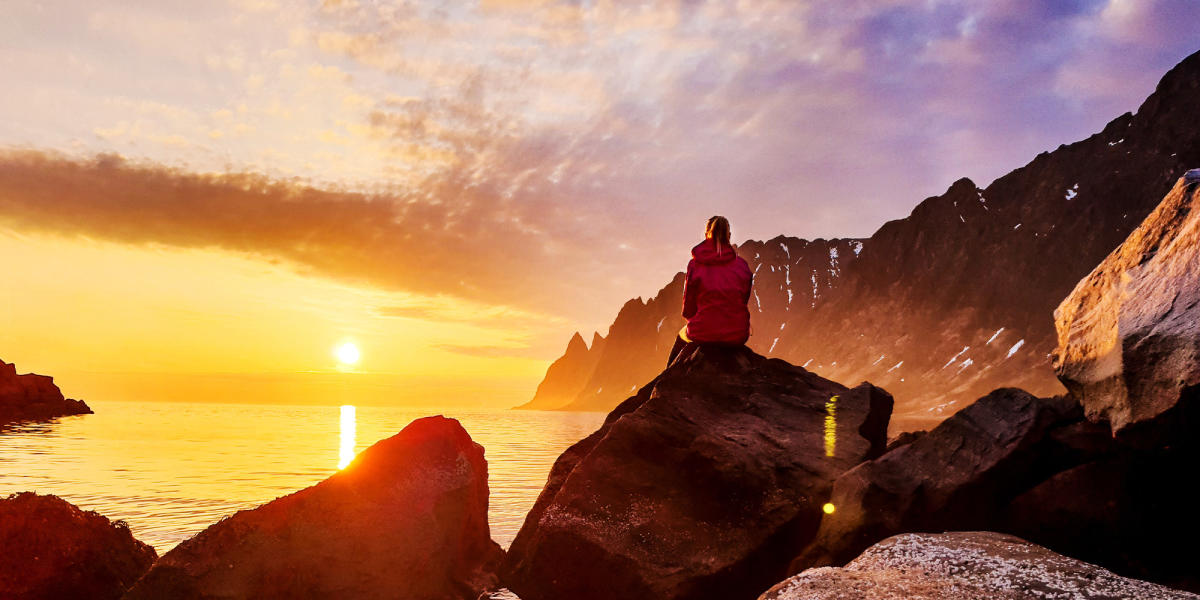In this rectangular photograph, a serene outdoor scene is captured during either a sunset or sunrise, with the longer sides of the image on the top and bottom. At the center of the image, the sun is positioned low on the horizon, casting a golden-orange hue across the sky and creating a striking contrast with the darker tones of the clouds above. These clouds, some dark gray, extend upward and across the sky, blending into bluish and purplish shades toward the right side. A vast and tranquil body of water stretches out from the foreground to the horizon, mirroring a brilliant line of sunlight that creates a path of reflected light on the water's surface.

In the foreground, there are several large, dark-colored rocks along the coast, with one particularly prominent rectangular rock in the center. Seated on the upper left point of this rock is a person, possibly a woman with long hair tied in a ponytail, wearing a red or purplish hoodie or jacket and black pants. Their leg is slightly visible, draped over the edge of the rock, and their posture suggests they are deeply engaged in observing the natural beauty before them.

To the right of this individual, more dark rocks appear, punctuated by a distinct white rock that seems to rise out of the darker formations. In the bottom right corner, a flat, brown rock with white and black spots partially extends out of the frame.

In the middle left of the image, a rocky land formation juts out into the water, leading the eye toward the horizon. The background showcases a majestic mountain range with peaks dusted in snow, stretching across the right side of the image and adding a rugged depth to the scene. Above, patches of gray clouds hover over these mountains.

Additionally, behind the person and to their right, there is a mysterious yellow light feature with what appears to be letters or symbols, adding an enigmatic touch to this otherwise tranquil and natural setting.